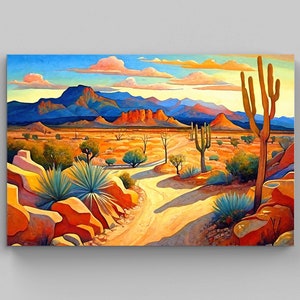The painting depicts a vibrant, sun-drenched desert scene on canvas, characterized by its striking use of color and rich, illustrative style. In the foreground, a winding sandy path stretches out, lined with yellow and orange rocks interspersed with yucca plants and small, spiky cacti. Succulents in shades of blue and green grow wild along the path. Tall cacti on the left cast heavy shadows, adding depth to the scene. As the path continues, it leads to clusters of small trees, indicative of the desert's arid conditions where large trees rarely thrive. In the background, the landscape unfolds into majestic red and orange mountains and cliffs, with blue-tinged mountains further along the horizon. Above it all, the sky is a brilliant blue with white clouds tinged yellow from the sunlight. The painting utilizes a masterful palette of bright blues, yellows, oranges, reds, and greens to create a vivid and almost surreal depiction of the desert, blending realistic elements with a distinctive illustrative vibe. The overall effect is both striking and beautiful, capturing the harsh yet enchanting essence of the desert landscape.